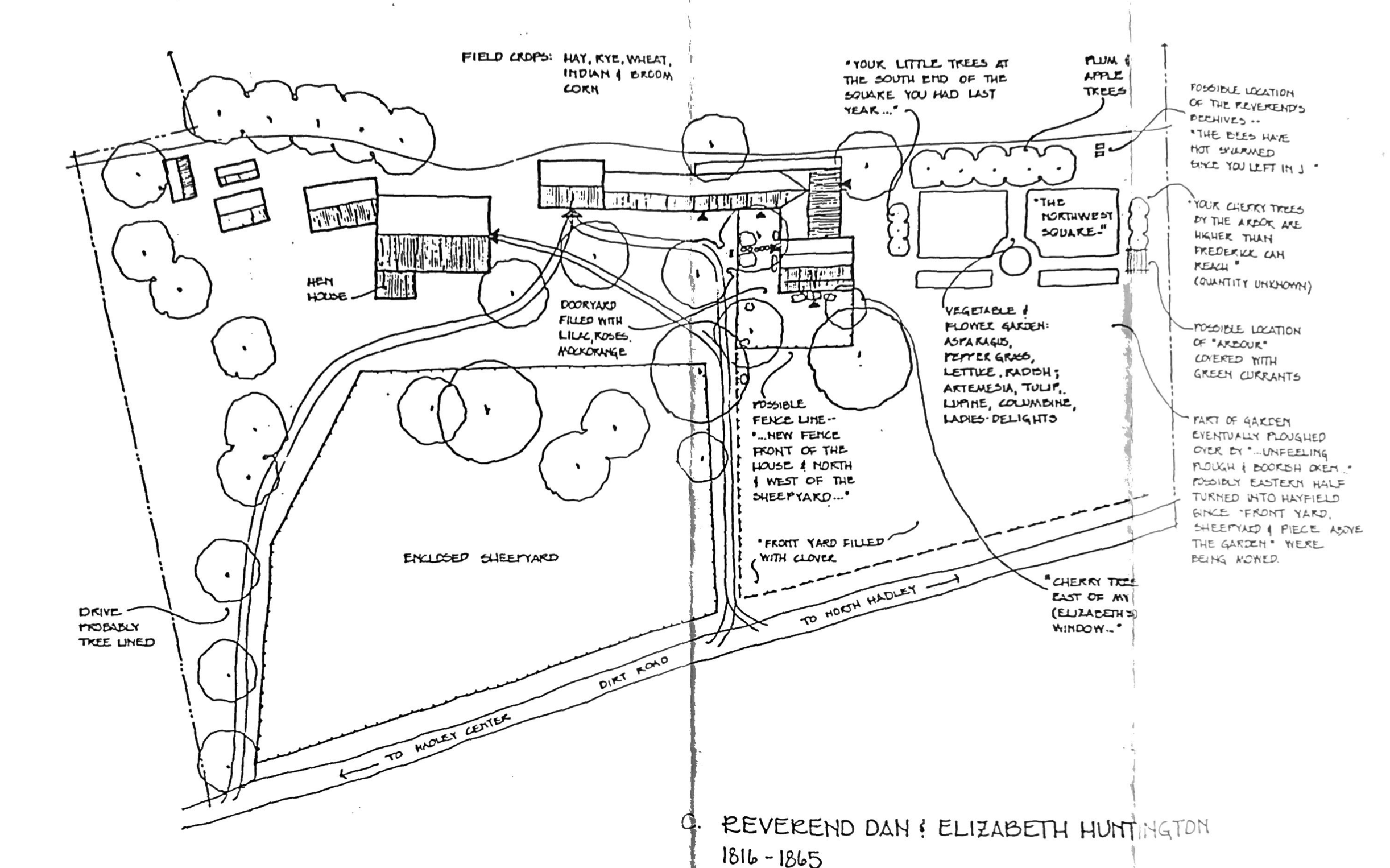This is a detailed, hand-drawn, black-and-white map of a small area, possibly a section of a town or a property layout, spanning from 1816 to 1865. At the bottom right, the map is titled "Reverend Dan and Elizabeth Huntington," with dates listed as 1816-1865. A road labeled "to North Hadley" runs diagonally from the bottom left to the center-right, while another area is marked as a "dirt road." The map is segmented into various labeled sections of land, including "enclosed sheep yard." Several labeled plots of crops such as hay, rye, wheat, and corn ("Indian") appear throughout the design. Additionally, areas labeled "Dooryard filled with lilac, hoses, and hawthorn" are indicated. The detailed layout captures the intended design and infrastructure of the property, complete with buildings and other land uses meticulously marked.